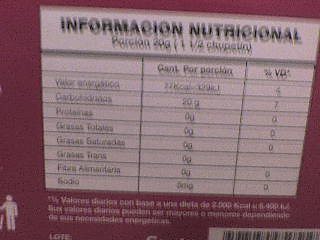The low-quality, landscape-oriented color photograph captures the nutritional information label on the back of a maroon-colored product package. The image is small and low-resolution, resulting in blurred text with noticeable grain and ghosting effects due to slight camera movement. The table, set against a white but off-colored background with black ink, contains three columns of data in Spanish, titled "Información Nutricional" at the top. The left column lists various nutrients, with "Carbohidratos" (Carbohydrates) and "Sodio" (Sodium) identifiable among them. The middle column, labeled "Por Porción" (Per Portion), shows nutritional values, with most entries reading zero grams. The right-hand side of the package features a black and white barcode, while the bottom left displays a white logo of a woman disposing of paper into a bin. The white balance of the image is off, further obscuring the details and making the text difficult to read.